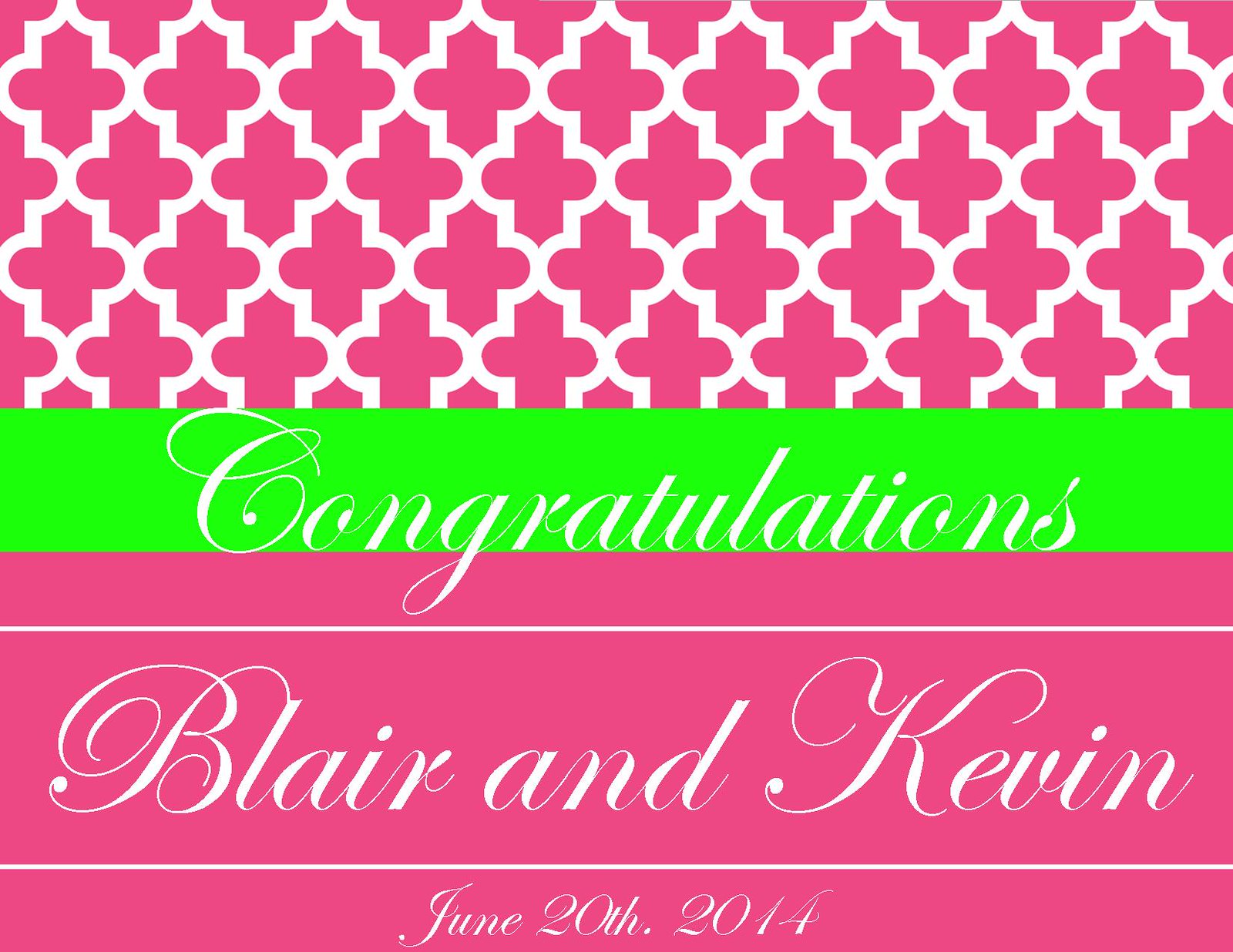The image features a vibrant and celebratory card that prominently uses shades of pink, green, and white. The top half of the card showcases a pink background adorned with intricate geometric patterns in white. In the center, a striking lime green bar displays the word "Congratulations" in white, italicized cursive. Below this central green bar, the pink background continues with a thin white bar separating the upper and lower sections. The bottom section features the names "Blair and Kevin" in elegant white italics and cursive, along with another white line below. Further down, the card also highlights the date "June 20th, 2014" in the same stylish font. The overall design suggests a vibrant and joyful occasion, possibly celebrating a wedding or graduation, with a bright and inviting aesthetic.